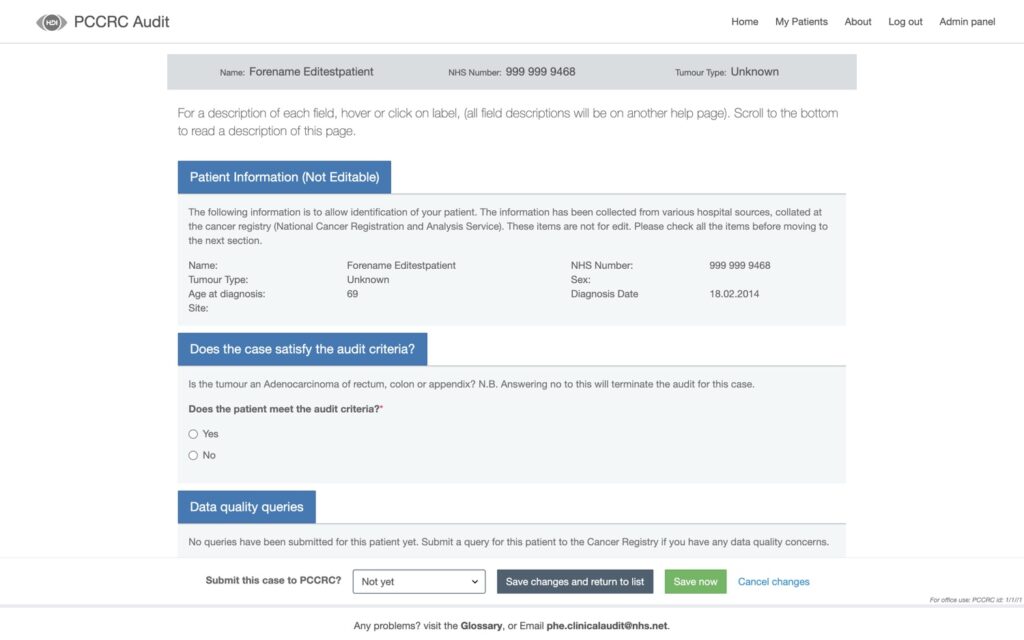**PCCRC Audit Portal Screen Capture**

The image is a screen capture from a specific website featuring a PCCRC (Post Colonoscopy Colorectal Cancer) audit. At the top, a gray circular icon with the initials "PCCRC" is visible, accompanied by a set of navigation options in gray text: "Home," "My Patients," "About," "Logout," and "Admin Portal." 

Below this, there is a thin gray bar labeled "Name" with the entry "Ed Test Patient." The NHS number is listed as 9999999468, and the tumor type is indicated as "Unknown."

A descriptive note follows: "For a description of each field, hover or click on the label. All field descriptions will be in another help page. Scroll to the bottom to read a description of this page."

Next, there is a blue box with white font labeled "Patient Information - Not Editable." This section clarifies that the information provided is for patient identification, collected from hospital sources and the National Cancer Registration and Analysis Service (NCRAS). The details in this section are not editable and should be confirmed before proceeding. The patient information includes:
- Name: Ed Test Patient
- Tumor Type: Unknown
- Age at Diagnosis: 69
- NHS Number: 9999999468
- Sex: Not listed
- Diagnosis Date: 18.02.2014

A query follows in a blue box with white font: "Does the case satisfy the audit criteria?" This is followed by an essential question in gray: "Is the tumor an adenocarcinoma of the rectum, colon, or appendix? Answering 'No' will terminate the audit for this case." There are two checkboxes for "Yes" or "No," both currently unchecked.

In the bottom section, another blue box with white font states "Data Quality Queries." It notes that no queries have been submitted for this patient yet and suggests submitting a query to the cancer registry if there are any data quality concerns.

Finally, there is an option to submit the case to PCCRC, which is currently marked "Not yet." Below this, additional options appear in a blue box with white font: "Save Changes" and "Return to List." Another green box with white font reads "Save Now," and a blue "Cancel Changes" option is also provided. 

At the very bottom, guidance is given for resolving any issues: "Any problems? Visit the glossary or email" followed by an email address.